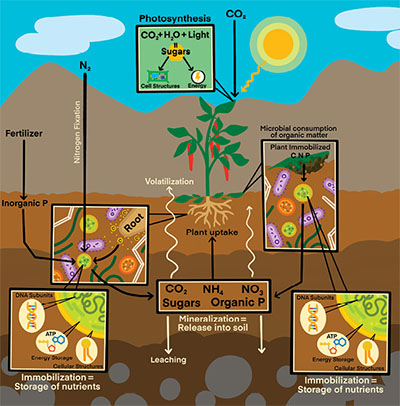The diagram illustrates the process of photosynthesis and nutrient cycles in plants, depicted in a cartoon style. At the top, a bright sun, symbolized by concentric circles in shades of yellow and orange, is labeled with "CO2" and has a black arrow pointing downwards. Positioned centrally, the diagram shows a green plant with red vegetables hanging from it. Above the plant, a box labeled "photosynthesis" explains that CO2, H2O, and light combine to form sugars, which are essential for cell structures and energy production. 

The diagram continues with various nutrient-related processes. On the left, brown mountains signify a natural environment, with arrows indicating fertilizer's impact on lighter soil labeled "inorganic P." Close-ups of microbes are shown, one labeled "root", and another section labeled "immobilization equals storage of nutrients," emphasizing nutrient storage within the soil. 

In the center, under the plant, is a breakdown labeled "plant uptake" demonstrating processes such as volatilization through a white squiggly arrow. A detailed close-up of soil shows a complex interaction of elements, including CO2, NH4, NO3, and organic P, highlighting the mineralization and leaching processes. 

On the right side, microbial activities are illustrated with labels like "plant immobilization C and P" and "microbial consumption of organic matter," showcasing how microbes contribute to nutrient cycling. Finally, various squares and rectangles portray nutrient storage, marking elements like DNA and ATP within the soil ecosystem. 

Overall, the diagram intricately details the interconnected processes of photosynthesis, nutrient uptake, and soil mineralization, emphasizing the flow and storage of essential nutrients within plant systems.